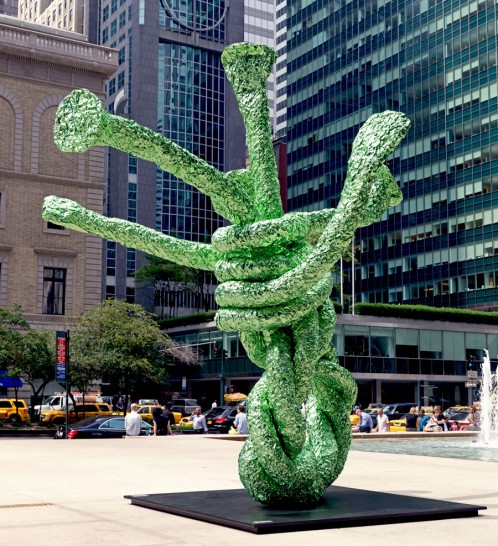This image captures a striking green and white statue set on a black platform in the bustling heart of a major city, possibly New York or Chicago. The sculpture, reminiscent of tangled vines or Medusa's snake hair, features intricate coils winding from the base to the top, with some of the coils uniquely resembling mushrooms. The profound deep green color of the statue contrasts sharply with its white accents. The scene is alive with urban energy, as numerous yellow cabs and cars move in opposite directions on the road in the center of the photo. To the right of the statue, a water fountain and small pool add a touch of tranquility amidst the busy atmosphere. The background is dominated by tall office buildings, traffic signals, and crowds of pedestrians, highlighting the city's vibrant and dynamic environment.